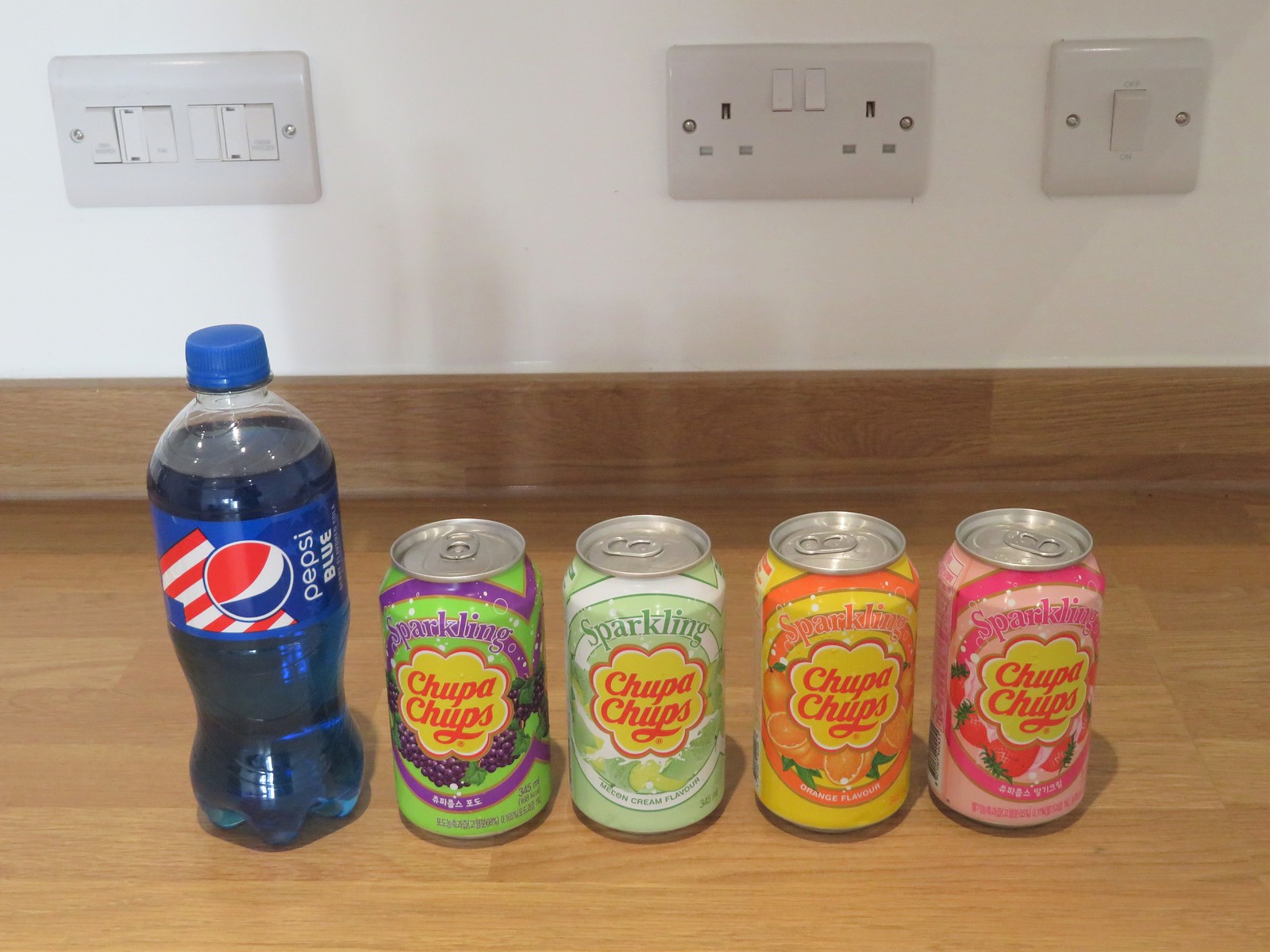The image depicts a section of a room with a white wall featuring a series of switches on both the left and right sides. There are three switches on the left panel and an additional set of switches on the right panel, possibly controlling various functionalities like lighting or blinds. Below the switches, there is a wooden baseboard, and the floor is constructed of yellow oak hardwood. Positioned on the floor, a small half-liter plastic bottle of Pepsi Blue is visible on the left side, notable for its blue liquid, blue cap, and a blue label adorned with the classic red, white, and blue Pepsi logo in a circle. Adjacent to the Pepsi bottle are four cans of Sparkling Chupa Chups, each with distinct flavors and vibrant colors. From left to right, the cans are as follows: a grape flavor featuring green and purple, a lime flavor in lime green and white, an orange flavor with orange and yellow, and a strawberry flavor in shades of pink and dark pink. All cans display the iconic yellow Chupa Chups logo with red lettering. The wooden countertop elevates slightly to meet the wall, creating a cohesive and detailed backdrop for the array of beverages.